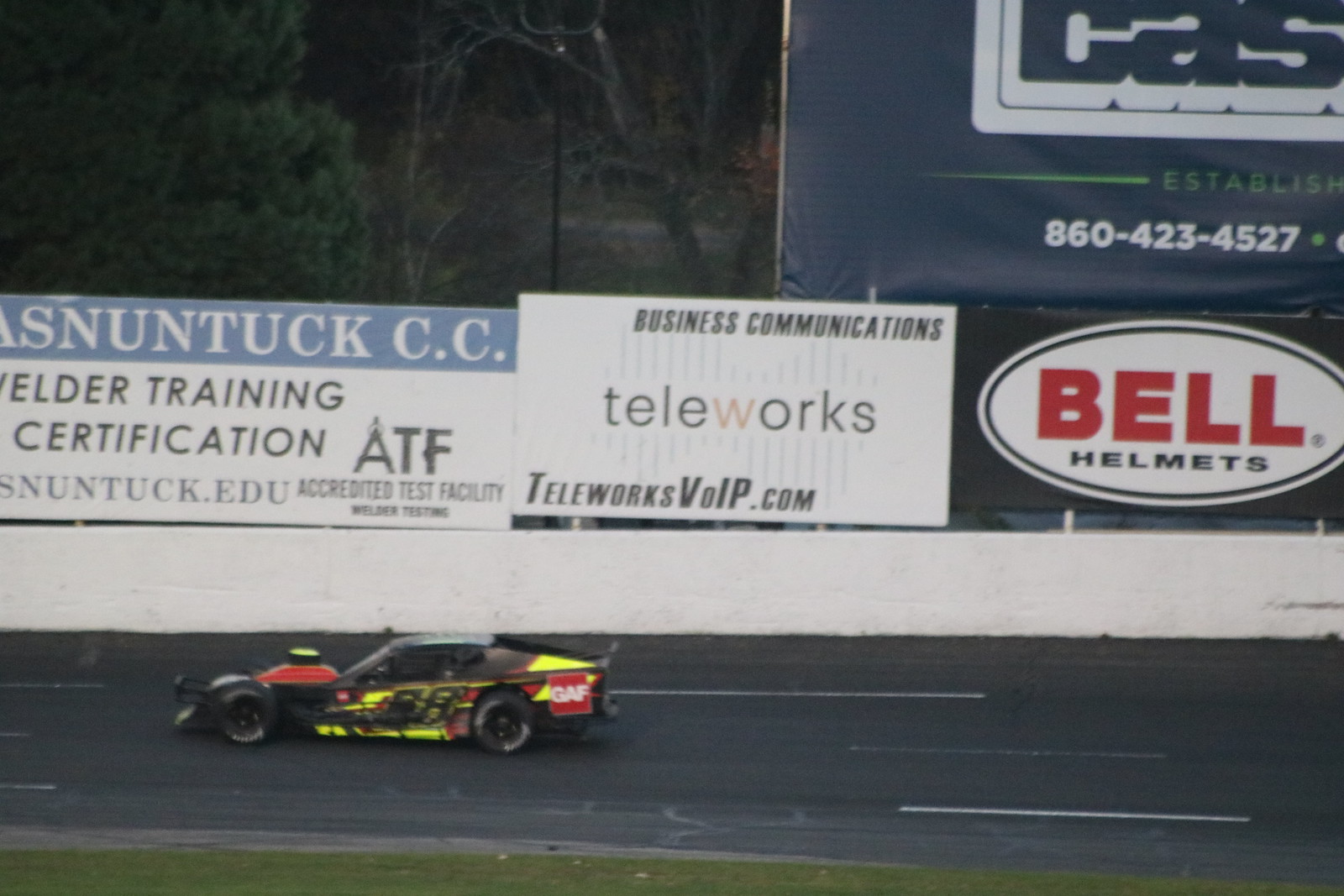The image captures a dynamic scene featuring a race car on a racetrack, surrounded by a vivid array of details. The race car, predominantly black with red and yellow accents, is positioned towards the bottom left of the image, racing along the black track marked with white stripes. The track runs horizontally from left to right, bordered at the bottom by a small patch of light green grass. Above the track, there's a protective white concrete wall adorned with multiple sponsorship signs.

The signs feature diverse advertisements, including Bell Helmets, Business Communications, Teleworks, teleworksvoip.com, Welder Training Certification, and ATF. These signs are a mix of white, black, light blue, dark blue, green, and red colors. Behind the wall, in the top left background, dark green trees are visible, adding a natural contrast to the man-made setting. The overall image conveys the thrill and motion of the race car in the middle of a competitive event, framed by vibrant advertising and lush greenery.